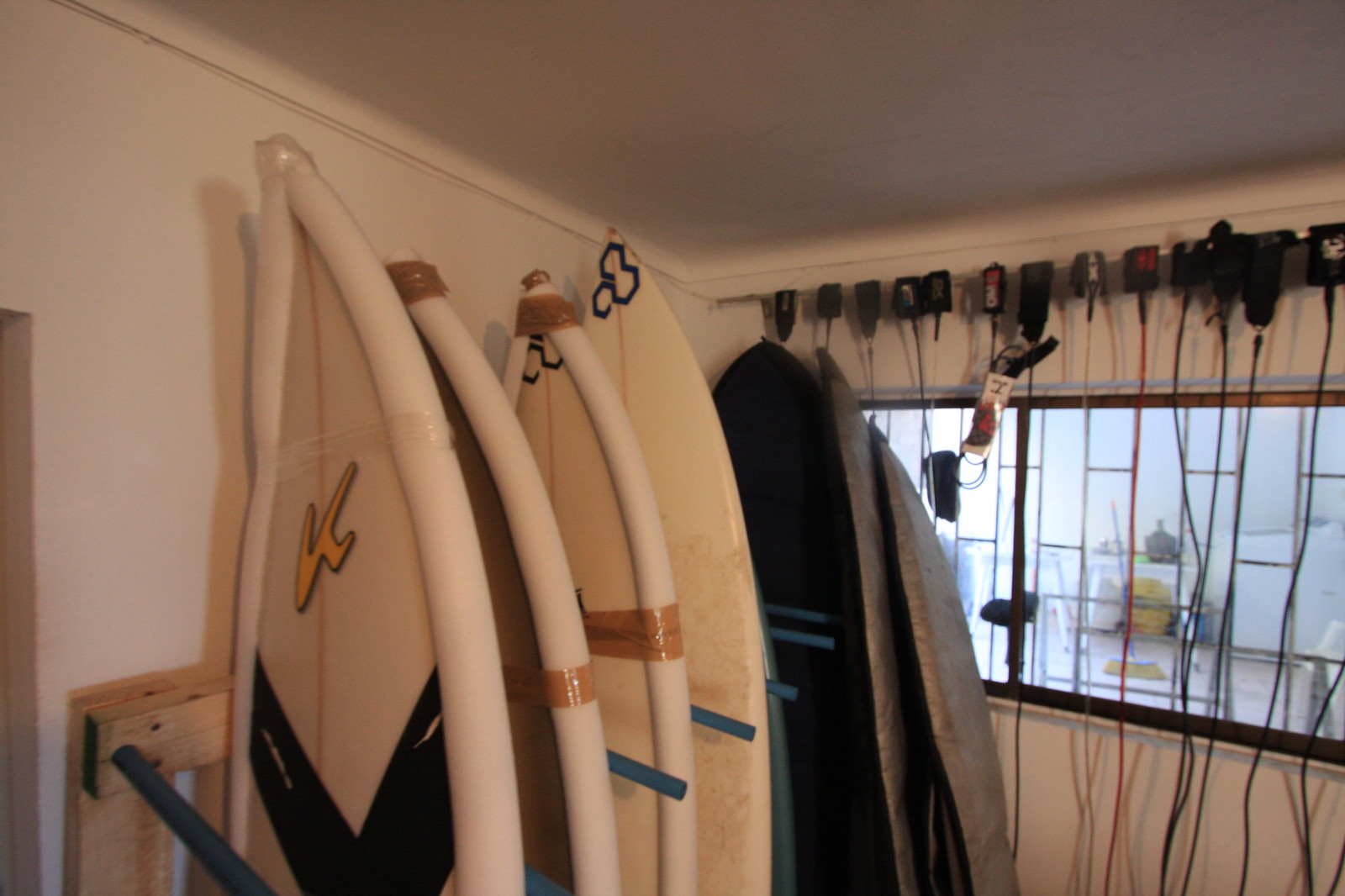The photograph captures an interior scene of a room, possibly a surf shop or a surfboard enthusiast's personal collection, painted in beige. The focal point on the left side of the room is a homemade wooden rack, constructed from 2x4s and black metal tubing, designed to hold surfboards. The rack’s tubing extends to the right, with blue separators and protective padding made of white foam or pipe insulation secured with packaging tape to protect the edges of the boards. There are six surfboards upright in the rack, primarily white with one or two darker, possibly black or dark brown, boards at the back. To the right, a black-framed, double horizontally sliding window with dark curtains hangs on the back wall. The room has a low ceiling and white walls, with additional details such as cords or curtain rods and surfboard leashes hanging above the window. The ambiance suggests either a rental setup or a personal surfboard storage area, brimming with a passion for surfing.